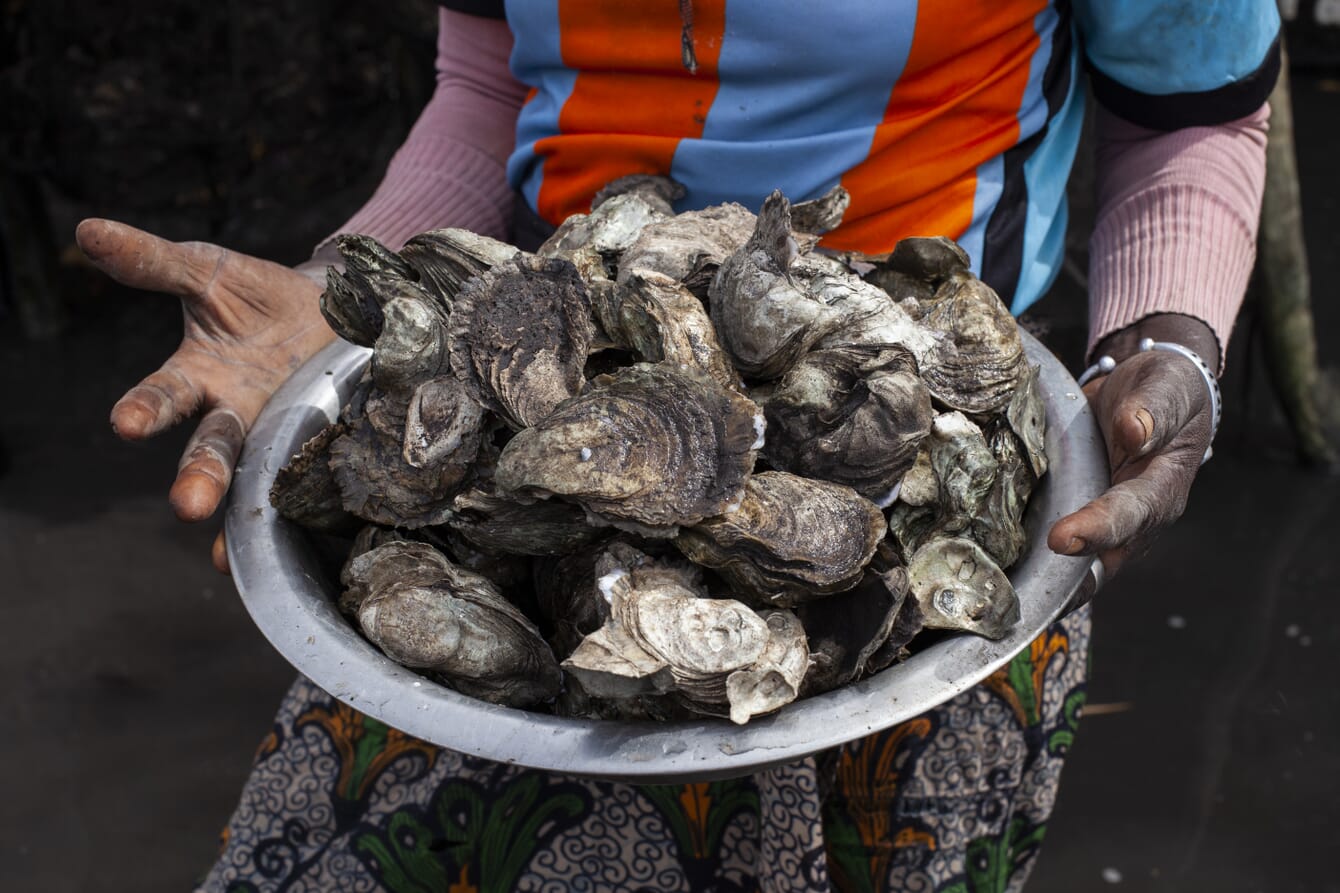In this photo, a woman with dark-colored skin is carrying a large, round silver bowl piled high with clams. The clams are notably dirty, still covered in dirt and gunk, giving them a ruddy appearance with different color variations. Some clams even seem to have a distinctive look, almost like one has a face with eyes and a nose. The clams are dry and their shells are still closed. The woman is seen from the chest down, dressed in a long sleeve pink sweater with a blue shirt featuring red stripes layered over it. She is wearing white pants decorated with black spirals and yellow, green, and orange flowers. On her right hand, she sports a silver bracelet, while her hands appear dirty with a white substance on them.